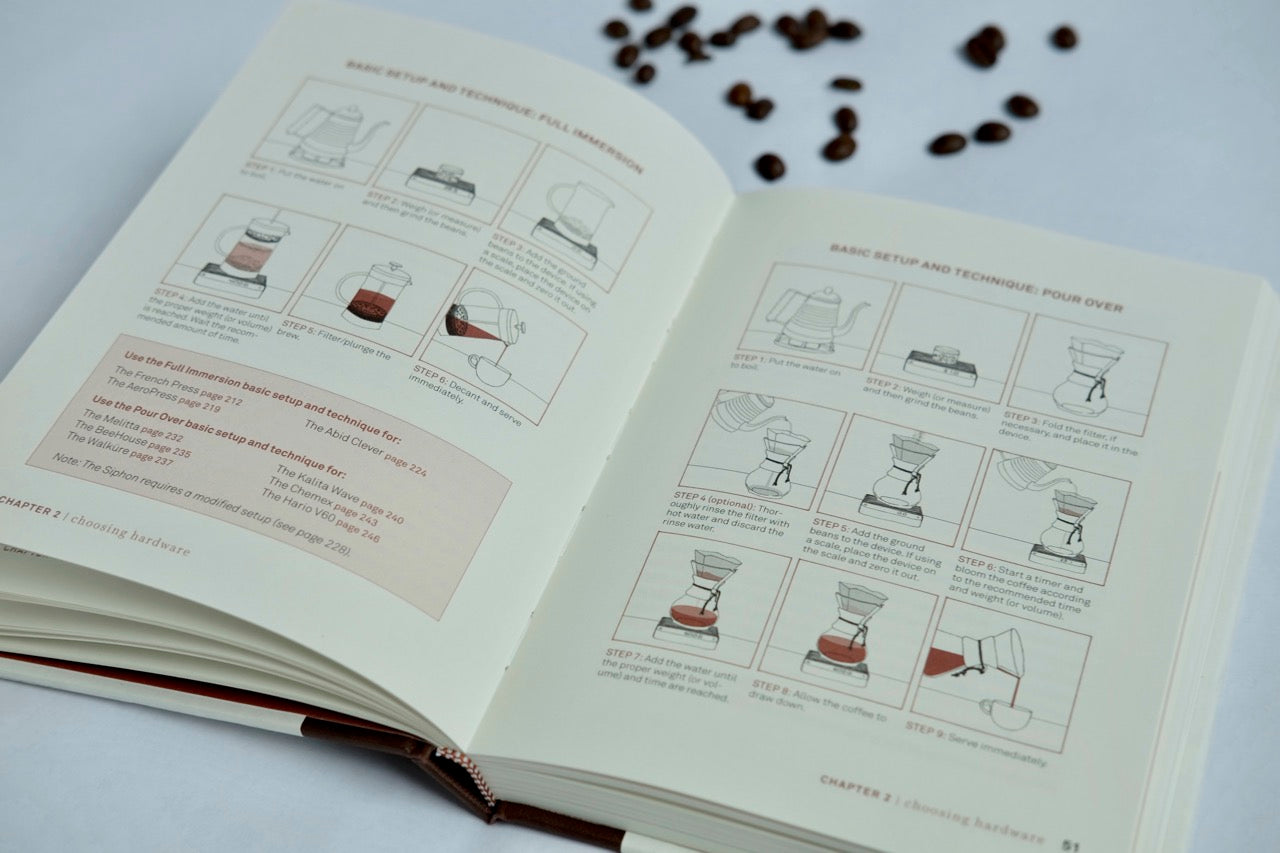This image shows an open hardcover book with a sewn spine, lying on a white surface with coffee beans scattered in the upper right corner. The book, possibly an advertisement for a comprehensive coffee brewing guide, is open to a page that demonstrates various coffee-making techniques. The left-hand page features six images, illustrating different steps involved in brewing coffee, including boiling water and pouring it over coffee grounds in a filter. A red box with red and black text is situated at the bottom of this page, though the writing is blurry and not legible.

On the right-hand page, the title "Basic Setup and Technique: Pour Over" is written in red at the top, followed by nine detailed diagrams that outline the pour-over coffee method. This involves boiling water, placing a coffee filter with coffee grounds, pouring the boiling water over the grounds, allowing it to drip through into a vessel, and then finally pouring the filtered coffee into a cup. The bottom of this page indicates it is Chapter 2 titled "Choosing Hardware," suggesting this book covers multiple coffee brewing methods, including other techniques like full immersion and French press, as hinted at in other sections. Overall, the book is structured to be a guide for various coffee brewing methods, complete with visual step-by-step instructions and detailed descriptions.